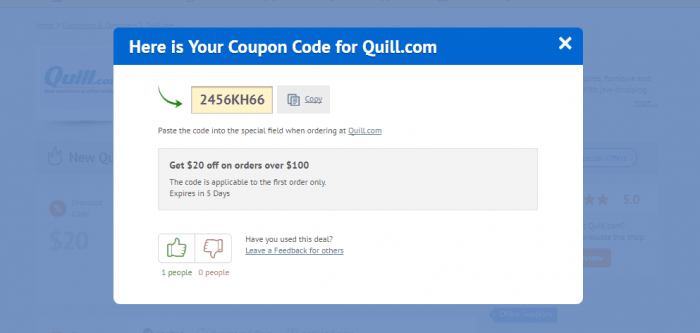The image is a horizontal screenshot featuring a central pop-up box on the Quill.com website. The pop-up box has a clean, white background and is topped with a blue banner that reads, "Here is your coupon code for quill.com." This banner includes an "X" on the right for closing the box. The overall background behind the pop-up is a translucent blue, allowing some of the text from the website to be faintly visible.

The pop-up box itself is outlined with a thin gray line and has a light yellow interior. Prominently displayed in the center is the coupon code "2456KH66," accompanied by a "Copy" button. Below this, there is an instruction that reads, "Paste the code into the special field when ordering at quill.com," with "quill.com" being an active link.

Further down, a light gray text box is inserted, stating, "Get $20 off on orders over $100. The code is applicable to the first order only. Expires in five days."

In the bottom left corner of the pop-up, there are two icons—a thumbs-up and a thumbs-down. The green thumbs-up icon is labeled with "1 people" in green text, while the red thumbs-down icon is accompanied by "0 people." To the right of these icons, a prompt asks, "Have you used this deal?" followed by a blue link inviting users to "leave a feedback for others."

Adding a touch of interaction, a small green arrow points towards the pop-up box, drawing the viewer’s attention to its contents.